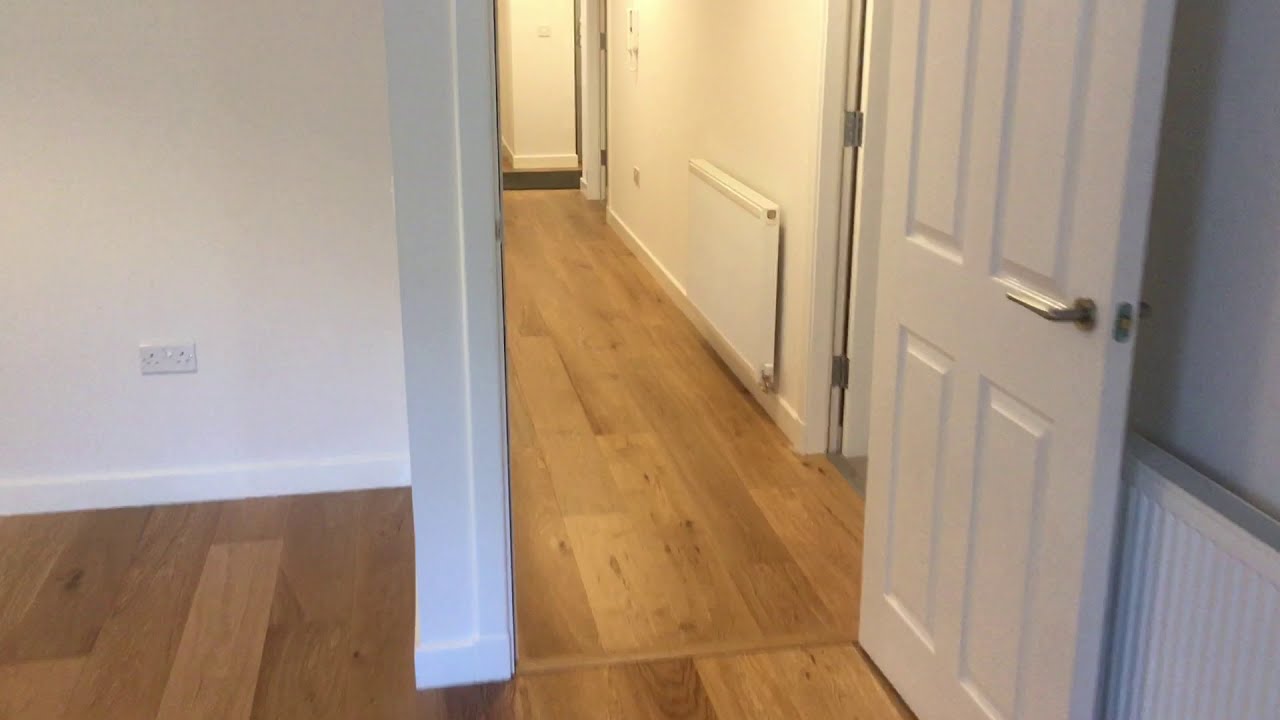This is an indoor photograph showcasing an empty house, potentially available for sale. The image is taken from within a room that opens into a hallway. The room and hallway feature light-colored hardwood floors, exhibiting a natural wooden pattern with visible tree knots. All the walls are painted white, providing a blank canvas throughout the home. The primary focus is on a white door, which is open and swings to the right. The door includes four large rectangular indentations and a gold handle. 

To the left of the room, a white electrical outlet is installed at the bottom of the wall. To the right, behind the open door, there is white lattice work against a gray wall with gray trim. The hallway extends in the middle of the image, lined with white walls and hardwood flooring, and opens to two additional rooms on the right side. Along the hallway, near floor level, a radiator can be seen. This clear and detailed image highlights the pristine and minimalist nature of the house’s interior, free of any text or people.